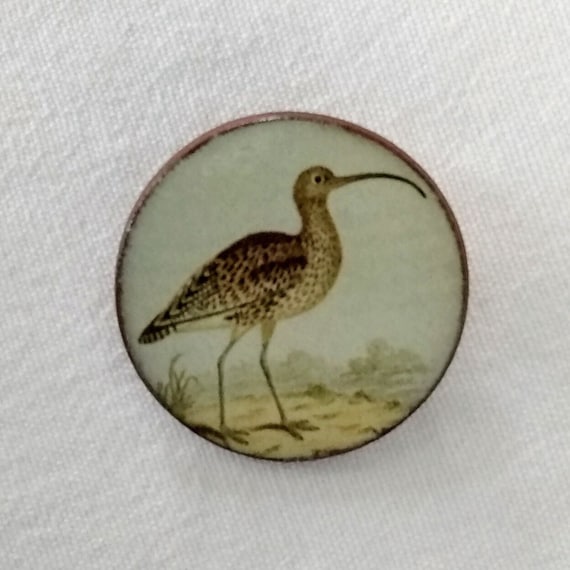This detailed image depicts a small, round painting or design centered on a white backdrop, possibly a tablecloth or napkin with visible seams. The artwork features a bird standing on a sand or desert-like surface with intermittent greenery, such as bushes. The bird is predominantly brown, with a dark brown body and white-speckled breast. It has a small head with a black eye and a notably long, curved black beak. Each of its two legs has three distinct toes. The bird's elongated wings and the black tip of its tail add to its distinctive appearance. The setting appears cold, contributing to the faded yet vivid portrayal of the scene. The round artwork is bordered by a brown edge, enhancing its detailed and compact nature.